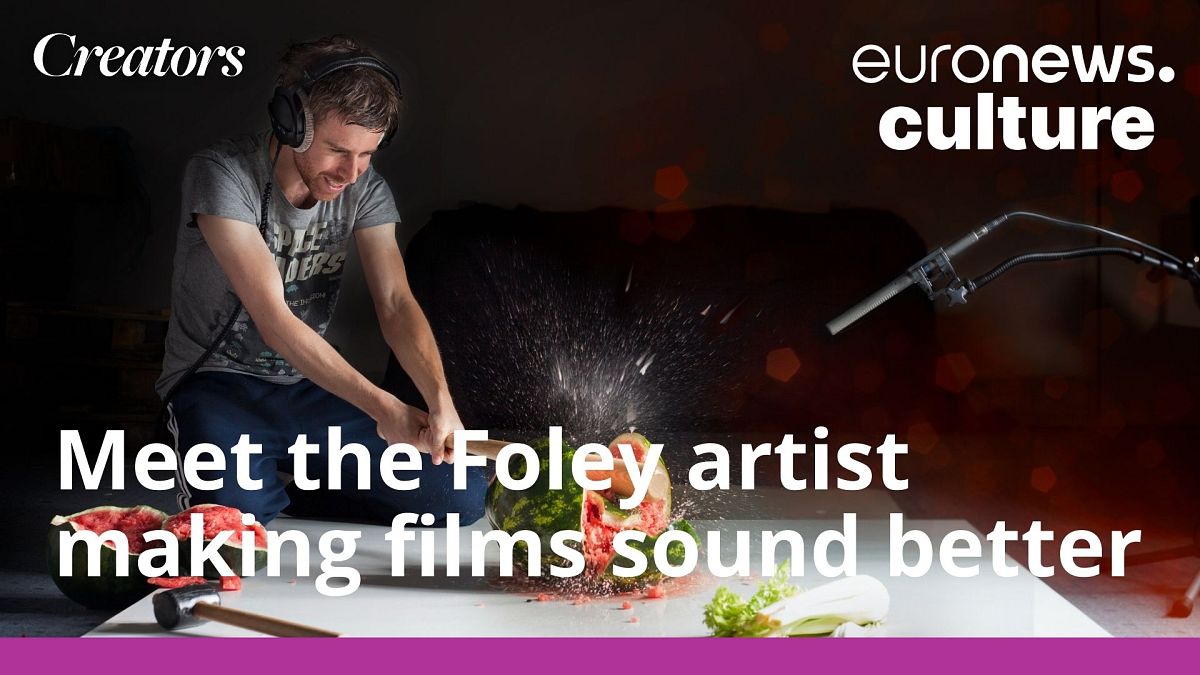The photograph features a man with dark hair, a mustache, and a well-trimmed beard wearing a gray t-shirt and blue jeans, kneeling on the left-hand side of the image. He is wearing headphones with a wire extending to his waist, and he holds a sword in his hand. The man has just sliced through a watermelon on a white table, causing it to split open and juice to fly into the air, revealing the pink flesh inside. Also on the table are other segments of watermelon, a sledgehammer, and possibly some longleaf lettuce. A large black microphone extends from the right side of the image, indicating that the sounds are being recorded. The background is predominantly black with a purplish-pink bar across the bottom. In bold white letters, it says "Meet the Foley Artist Making Film Sound Better" at the bottom of the image. In the top left corner, "Creators" is written in white, and in the top right corner, it says "Euronews Culture" in white letters. The scene captures the intricate work of a Foley artist producing sound effects for films or TV shows.